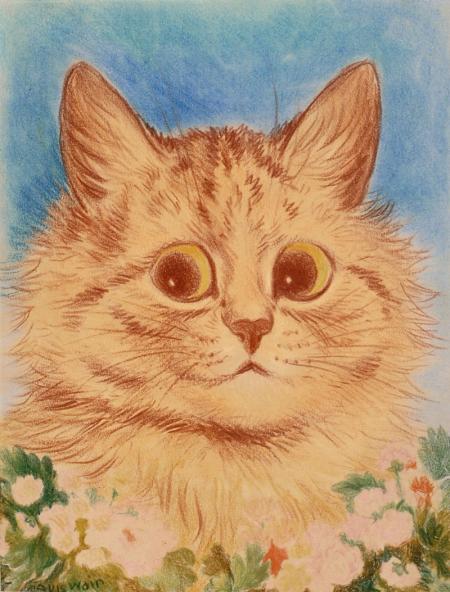This image depicts a detailed and realistic colored pencil sketch of a large-faced cat with extraordinarily wide, dark yellow eyes that gaze off to the side. The fur of the cat is predominantly beige with pronounced black, tiger-like stripes along its forehead and under its chin. Its ears are erect and shaped like inverted V's, complementing the dark whiskers that frame its face. The feline is the focal point of the image, occupying the central portion, while a vibrant blue sky with white clouds forms the background. Beneath the cat, there are various white flowers with green leaves, adding to the natural setting. The artist's signature is faintly visible in the lower-left corner but is not entirely legible. The composition as a whole is highly detailed and skillfully executed, emphasizing the cat's striking appearance and expressive eyes.